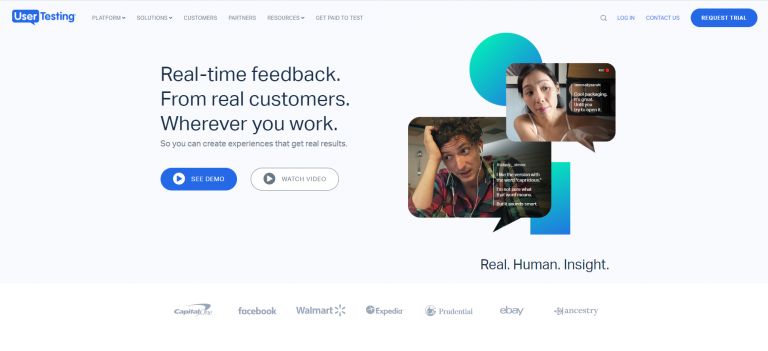The webpage prominently features the UserTesting logo at the top left corner, with "User" displayed in white text inside a black quotation box and "Testing" in blue text inside a blue quotation box. Along the top of the page, a gray navigation bar includes various options: Platform, Solutions, Customers, Partners, Resources, and Get Paid to Test.

Central to the page, a bold headline reads "Real-time feedback from real customers wherever you work," with a subheading in smaller text that extends the message: "So you can create experiences that get real results." Below this text are two call-to-action buttons. The first button, in blue, prompts visitors to "See Demo," while the second button, in white, invites them to "Watch Video."

To the right of this central section, there are images of two different individuals, each in their own quotation box, wearing headphones and seemingly engaged in a conversation. Although the accompanying text is too small to read, it is present on the page. These images are accentuated by blue shapes, including one circle and one rectangle, that add a visual element to the design. Beneath these images, a caption reads "Real human insight."